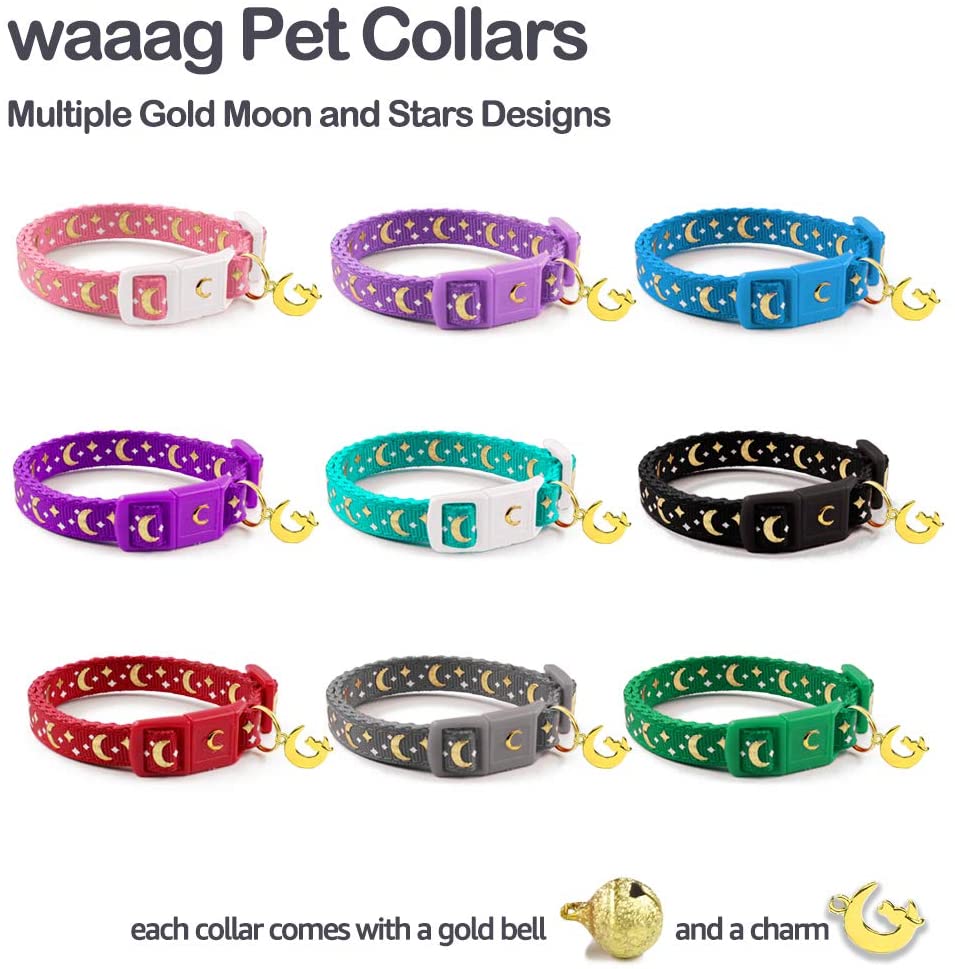This image is an advertisement for WAG pet collars, spelled W-A-A-G, which features prominently in large black lettering at the top. Below this, smaller text reads "multiple gold moon and stars design." The image displays a grid of nine pet collars, each featuring gold moon and star patterns and a dangling gold charm of a crescent moon with a cat sitting on it. The collars come in nine colors: pink (with a white buckle), light lavender, blue, darker purple, teal (with a white buckle), black, maroon, gray, and green. The buckles of the collars generally match their respective collar colors, except for the pink and teal ones which have white buckles. At the very bottom of the image, a note informs that each collar comes with a gold bell, depicted in a small picture alongside the description, and the crescent moon charm.